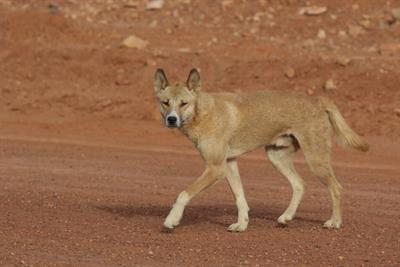In this striking desert scene, a wild dog, possibly resembling a wolf, strides across red, clay-like sand speckled with brown and reddish rocks under a bright, clear sky. The dog is light brown with a sleek, unfluffed coat clinging to its body, accentuated by lighter hues and almost white "sock-like" paws. Its fur transitions to an even paler shade around its muzzle and black nose. The dog is captured mid-step, moving from the right side of the frame to the left, its fluffy tail hanging down but slightly uplifted at the end. Its sharply alert, narrowed eyes and perked ears give it a vigilant look as it gazes directly into the camera, casting a stark shadow on the gravelly desert floor.